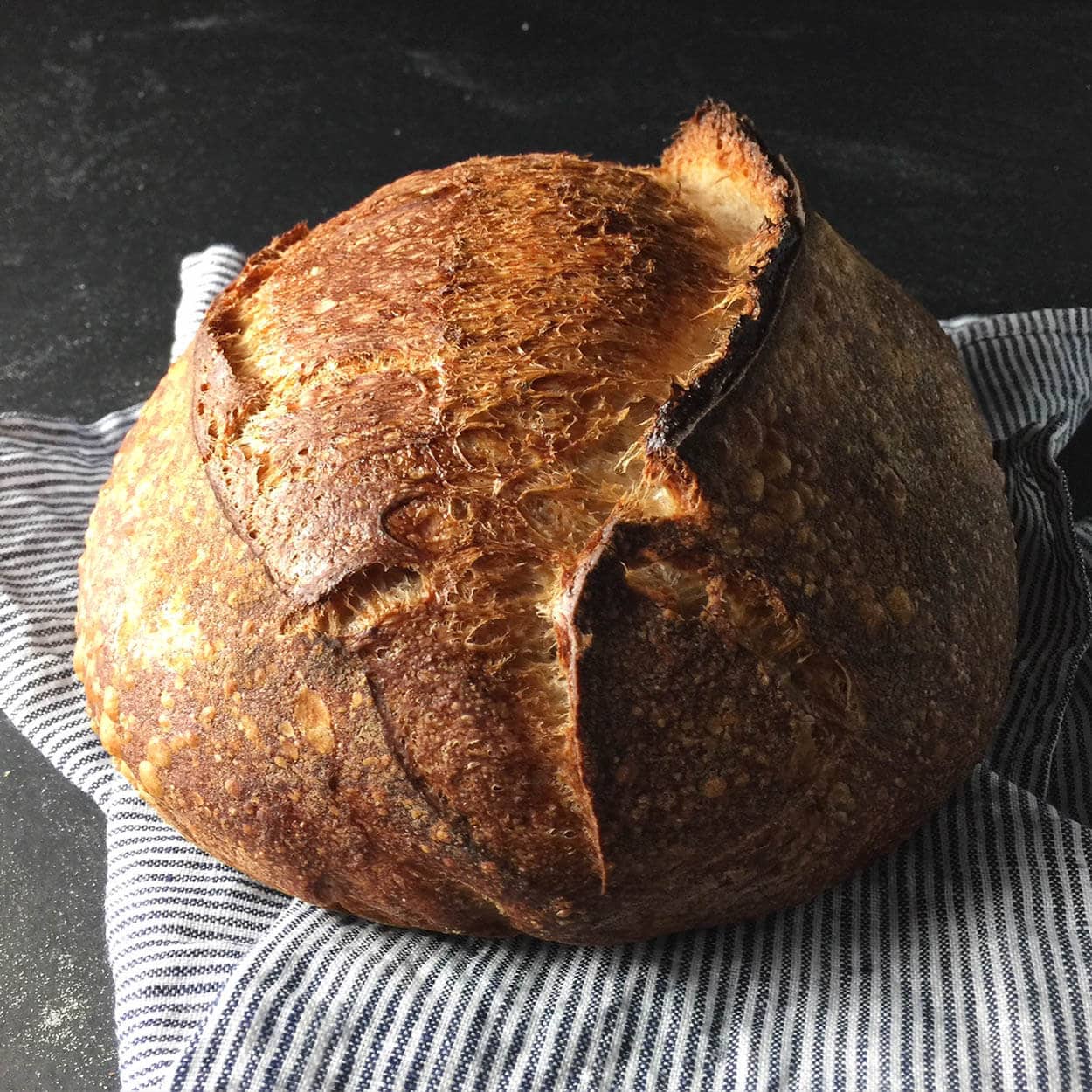This color photograph features a large, artisanal, football-shaped loaf of bread, freshly baked and fully intact. The outer crust is a deep brown, with some sections featuring near-black charring, indicative of a well-done bake. The loaf’s dome-like top is ridged, with some areas having a slightly burnt, blackened appearance, giving it a rugged, homemade look. The bread rests on a thin, pinstriped kitchen cloth with white and blue stripes, itself laid atop a dark gray stone slab. The overall presentation emphasizes the rustic, hearty nature of the bread, suggestive of a traditional, handcrafted baking process.